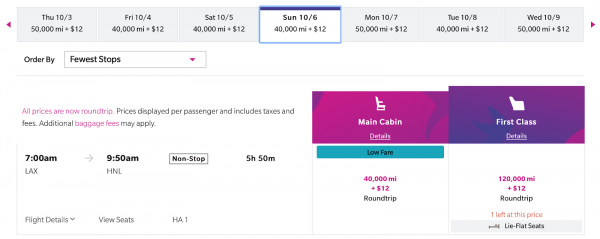This section of a webpage showcases flight booking details, notably highlighting a specific non-stop flight from LAX to HNL on Sunday, October 6, priced at 40,000 miles plus $12. 

At the top of the webpage, there are seven date entries: 
- Thursday, October 3 (50,000 miles, $12),
- Friday, October 4 (40,000 miles, $12),
- Saturday, October 5 (40,000 miles, $12),
- Sunday, October 6 (40,000 miles, $12),
- Monday, October 7 (50,000 miles, $12),
- Thursday, October 10 (40,000 miles, $12),
- Wednesday, October 9 (50,000 miles, $12).

The highlighted flight on Sunday, October 6 shows as follows:
- Departure: 7:00 AM from LAX (Los Angeles International Airport).
- Arrival: 9:50 AM at HNL (Honolulu International Airport).
- Duration: 5 hours 50 minutes, non-stop.

The webpage features options to filter flights by "Fewest Stops" with a drop-down menu. It informs users that all prices are for round trips, have possible delays per passenger, include taxes and fees, and that additional baggage fees may apply.

For the highlighted flight, there are further details under "Flight Details" and "View Seats". Users can choose between two cabin options:
- Main Cabin: 40,000 miles plus $12, including low fees, round trip.
- First Class: 120,000 miles plus $12, round trip, with one seat left at this price, featuring live flat seats for extra comfort.

The top banner of the page reiterates the available flights and prices for the range of dates listed.